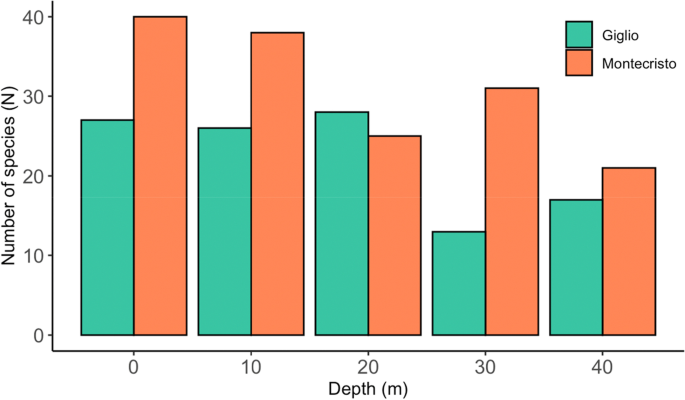The image depicts a computer-generated bar chart comparing the number of species between two locations: Giglio and Monte Cristo. The bars are colored seafoam green for Giglio and orange for Monte Cristo, as indicated in the legend at the top right of the chart. The y-axis, labeled "Number of Species," ranges from 0 to 40 and is marked in increments of 10. The x-axis, labeled "Depth (m)," also ranges from 0 to 40 meters, marked in similar increments.

There are five columns, each representing a different depth: 0, 10, 20, 30, and 40 meters. For each depth, there are two bars; the seafoam green bar for Giglio is positioned to the left, followed by the orange bar for Monte Cristo. Generally, the number of species decreases with increasing depth, and Monte Cristo often has a higher number of species than Giglio, except for one instance where Giglio outnumbers Monte Cristo.